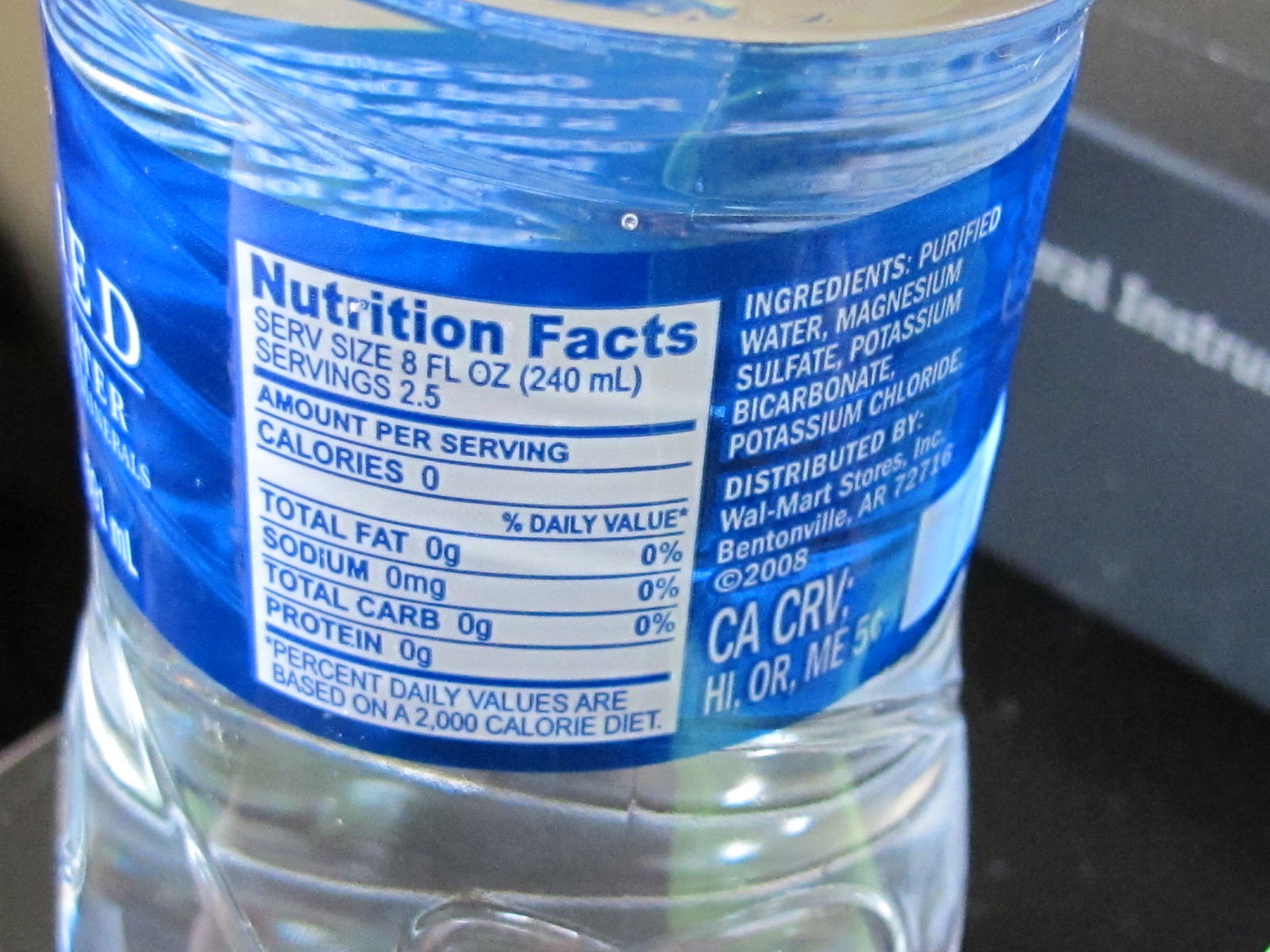This detailed close-up photograph highlights a plastic water bottle's label, with the main focus on the Nutrition Facts box. The clear bottle features a blue label wrapping around its circumference. The central white Nutrition Facts box, adorned with blue text, specifies a serving size of 8 fluid ounces (240 millilitres) and notes that the bottle contains 2.5 servings. Adjacent to the Nutrition Facts, the ingredients list—displayed as white text on a blue background—states the contents: purified water, magnesium sulfate, potassium bicarbonate, and potassium chloride. Below the ingredients, the label details the bottle's distributor as Walmart Stores, Inc., based in Bentonville, Arkansas (zip code 72716) and marks the copyright year as 2008. The photograph, taken on a dark surface, shows the reflective quality of the bottle and includes a note on the label indicating a cash value of five cents.